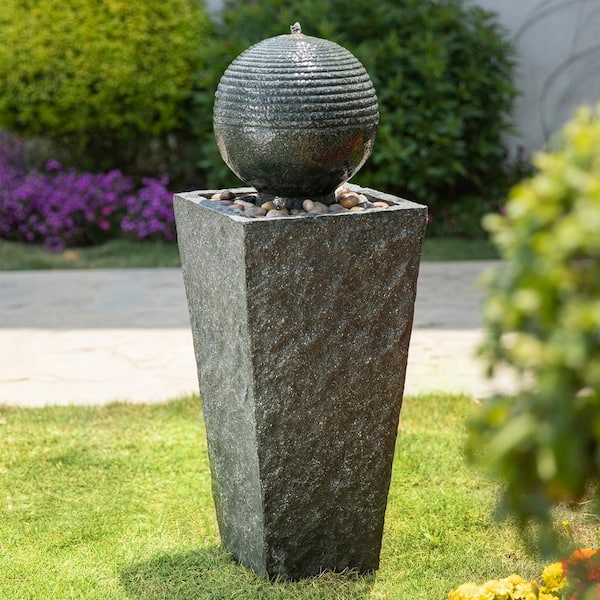The image features a detailed stone sculpture situated on a green grass lawn. The sculpture consists of a four-sided stone pedestal that widens as it rises. The top of the pedestal is filled with gray, white, and tan river rocks. Resting atop these rocks is a metallic, planet-like sphere adorned with circular ridges on its upper half and culminating in a small, pointed nub, possibly silver in color. Behind the sculpture, a gray walkway meanders through the garden, which is adorned with green bushes and vibrant purple flowers. To the right of the sculpture, a large green shrub with broad leaves stands out, while in the background, additional bushes and flowers add to the garden's serene ambiance.